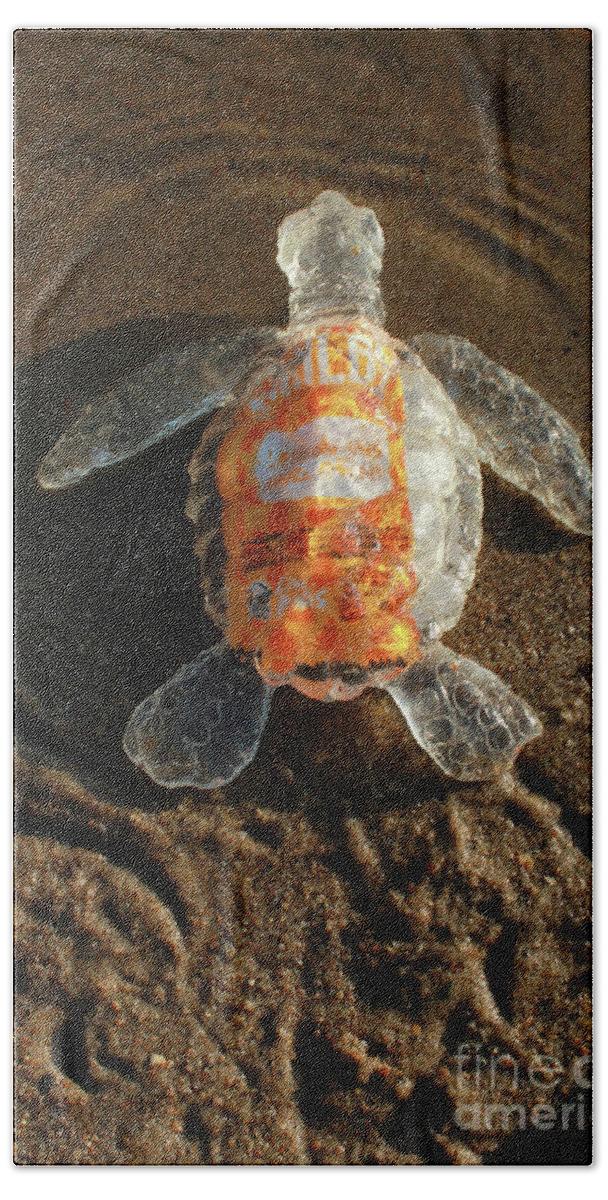This intriguing and surreal photograph captures a translucent sea turtle, remarkably crafted to resemble glass or clear plastic. The turtle's body, including its flippers and head, shines with a glassy, see-through quality, emphasizing a stark departure from reality. From a rear-view perspective, the turtle's shell prominently features an unusual orange and white object, which closely resembles a label or a sauce packet, possibly from a fast food brand like Taco Bell. The text on this label is illegible, adding to the mystique. The turtle is positioned on wet, sandy beach terrain, seemingly making its way toward the water, creating subtle ripples where its body meets the edge. The photograph, which appears grainy and aged, may have originated from a magazine or newspaper, as evidenced by halftone patterns and creases. In the lower right corner of the image, the text "Fine Art America" is partially visible in white, suggesting an artistic or commercial classification of the scene. This striking blend of elements delivers a powerful commentary on environmental issues, juxtaposing nature with artificial objects.